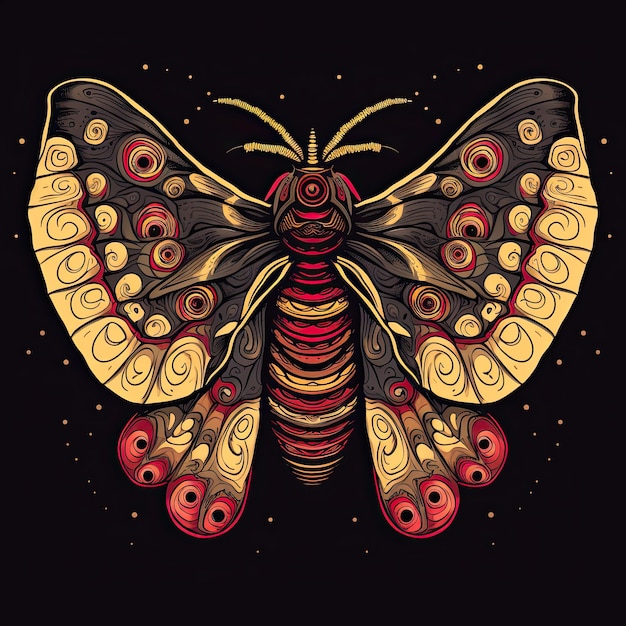This is an intricate illustration of a large, visually striking butterfly set against a black background adorned with tiny gold dots scattered throughout. The butterfly, which dominates the composition, features exquisite wings edged in gold with additional smaller gold designs moving inward. The outer edges of the wings resemble the shape of large toes or fingernails and are primarily yellow with a swirly pattern. Each wing is detailed with reddish-pink and gold circular designs, some containing black dots that give an eye-like appearance. The butterfly's body showcases horizontal stripes in red, gold, and black, creating a vibrant pattern that extends from its tail to its head. The head is quite unique, appearing to wear a gold mask with black detailing that resembles an open mouth and evil eyes, and adorned with gold tentacles reminiscent of dreadlocks or leaves. The butterfly's aesthetic hints at a carefully crafted, computer-generated image, blending elements of traditional drawing with digital precision.